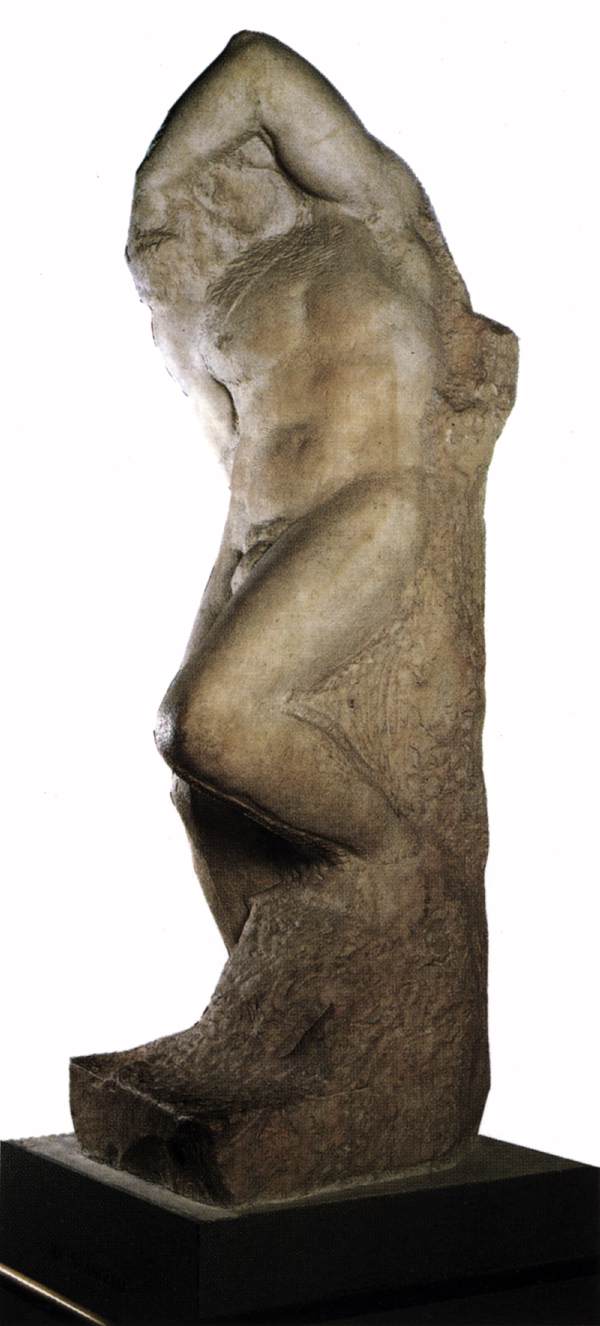The image showcases a detailed sculpture of a man, crafted to evoke the classical art of ancient empires such as the Ottoman Empire. The sculpture appears to be made from a dark gray or iron-hued marble, while the pedestal is black. The figure is intricately sculpted, partially emerging from what looks like a large, rough stone slab. The left profile of the man is prominently on display: his well-defined chest and abdomen leading to a bent left leg. His feet are not visible, possibly embedded in the stone. The man's left arm extends upward, covering his head and partially obscuring his face, creating an upside-down V shape. His head is slightly tilted to the side, with discernible hair details. This pose may suggest a theme of entrapment or transformation, reminiscent of mythical tales where individuals turn into stone, adding a layer of ancient mystique to the scene.